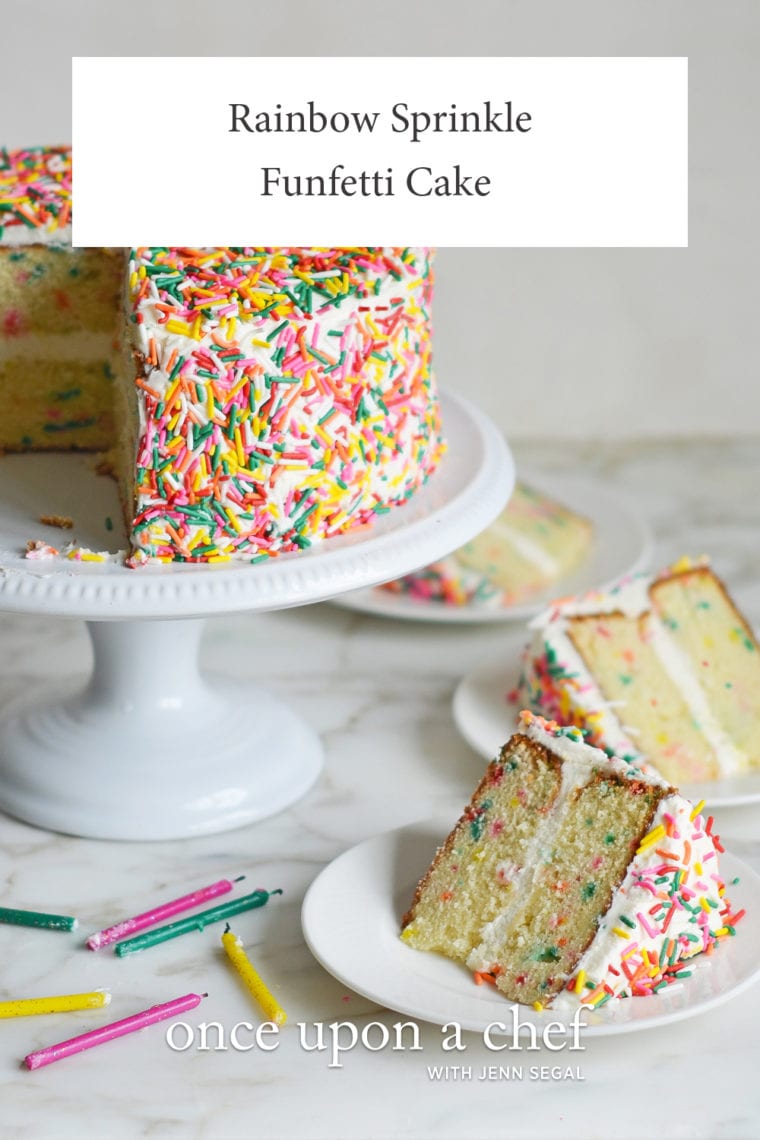This enticing photograph, potentially the cover of a cookbook titled "Once Upon a Chef with Jen Seagal," showcases a visually appealing Rainbow Sprinkle Funfetti Cake. The cake, presented on a pristine white cake stand with a circular base, is missing about a quarter slice, revealing its moist, yellow interior speckled with colorful funfetti. The cake is adorned with multicolored sprinkles in hues of yellow, white, pink, red, and orange on a smooth white frosting. Set on a white background, the scene is complemented by the blue-lettered sign above that reads "Rainbow Sprinkle Funfetti Cake." Surrounding the main cake, three white plates each hold a generous slice, ready to be savored. Scattered around are six blown-out birthday candles in pairs of pink, yellow, and green, with some even dotted with frosting remnants. The vibrant colors and inviting presentation of this cake make it irresistible, capturing a festive mood perfect for a celebration.